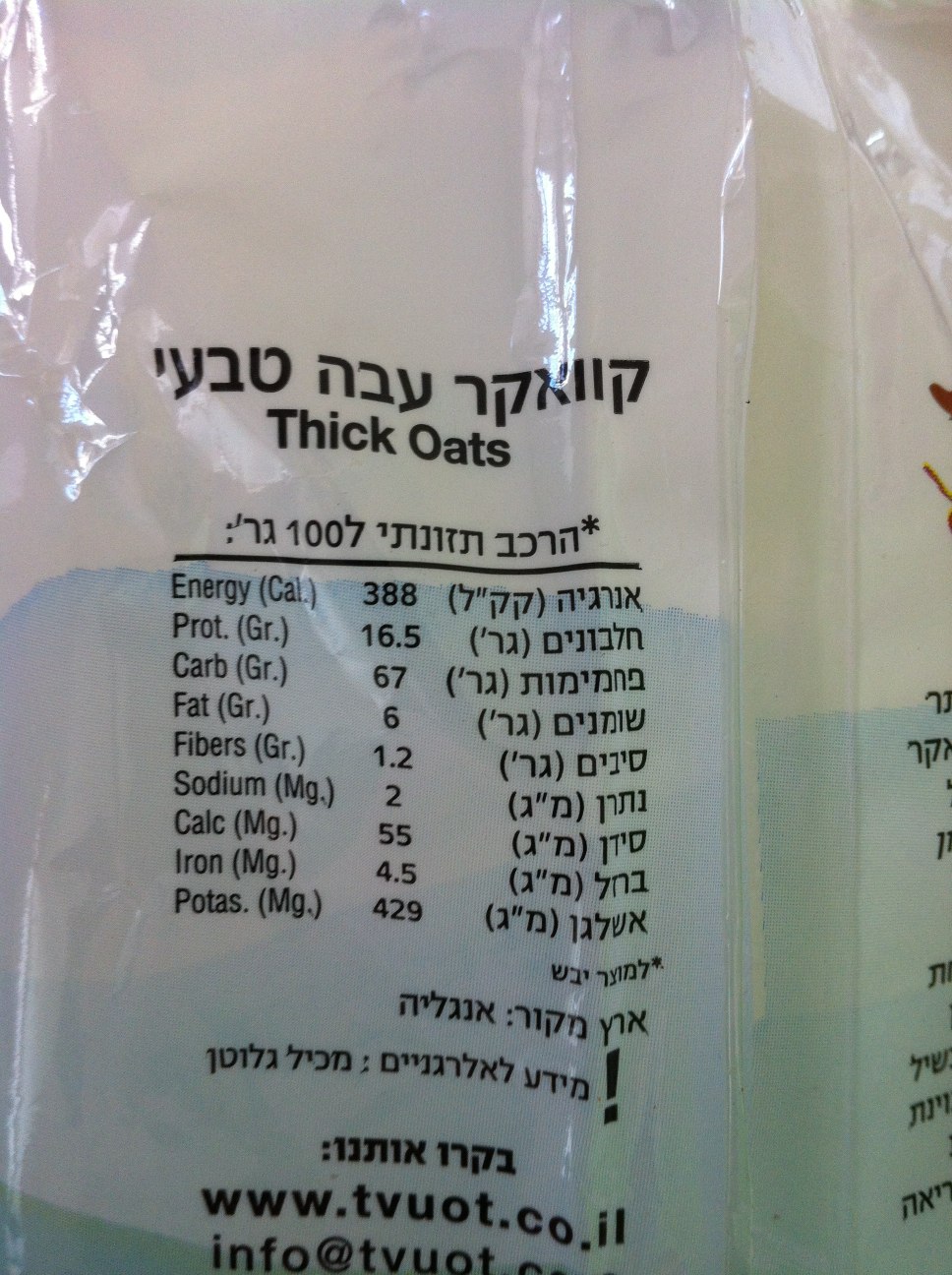This photograph captures a close-up view of the nutritional label on a package of thick oats. While the packaging predominantly features text in Hebrew, several key nutritional terms appear in English. These terms include "energy," "protein," "carb," "fat," "fibers," "sodium," "calc," "iron," and "potass." The detail of the thick oats imagery and the bilingual text hints at an international product, likely catering to both Hebrew and English-speaking consumers. At the bottom of the package, the website www.tvuot.co.il is visible, reinforcing the indication that this product originates from a Hebrew-speaking region, likely Israel. The combination of the descriptive nutritional information and the bilingual packaging offers an insightful glimpse into this health-conscious food product.